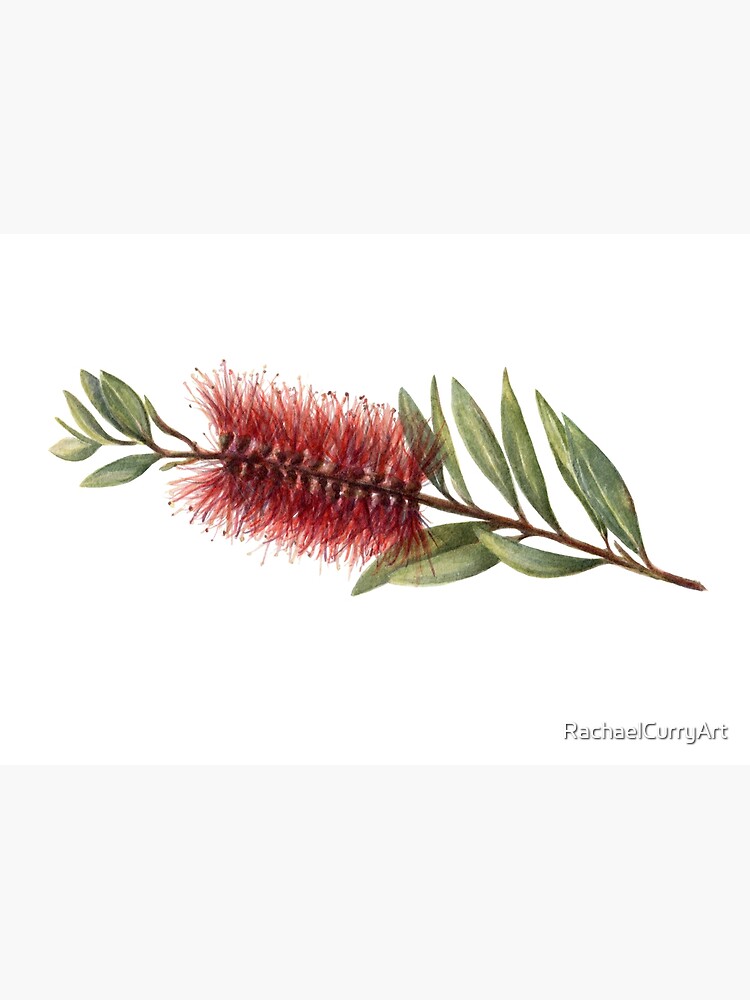The image portrays a watercolor painting or drawing by Rachel Curry, as indicated by the signature "Rachel Curry Art" at the bottom right corner. Set against a white background with two grey bezels above and below, the artwork features a brown twig adorned with several green leaves, both at the top and bottom. The leaves are slender and pointed, resembling arrowheads. Prominently, the twig is adorned with red filaments, clustered together in a manner reminiscent of a bottle brush, adding a striking contrast to the greenery. The painting's intricate details and simple palette underscore its delicate and naturalistic aesthetic.